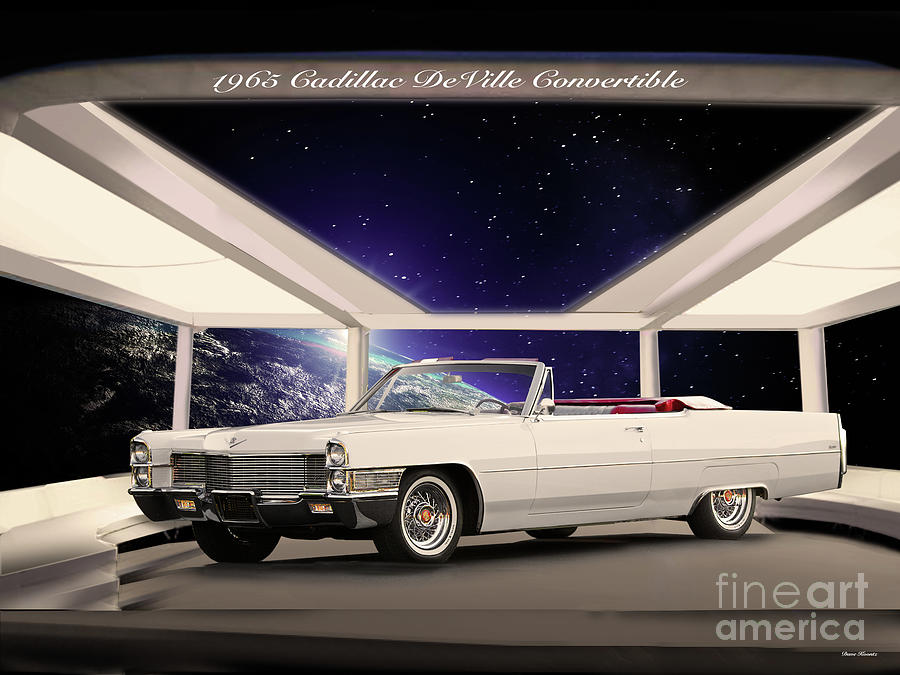The image showcases a sleek, white 1965 Cadillac DeVille Convertible positioned on a gray platform. The car's sophisticated design is emphasized by its chrome metal grille, silver rims with red detailing, and a luxurious interior featuring red and gray upholstery alongside a black steering wheel and gray mirror. The Cadillac, with its top down, enhances the scene's open feel. Above the car, in white cursive text against a brown stripe, is the model's name: "1965 Cadillac DeVille Convertible." The backdrop merges art and fantasy, depicting a celestial scene with a prominent view of Earth, its blue and white hues mingling with lighter shades and a hint of pink, set against a black sky studded with white stars. The entire composition, spanning multiple visual elements, is further enriched by a subtle acknowledgment of its artistic origin, labeled "Fine Art America" in gray text at the bottom right.